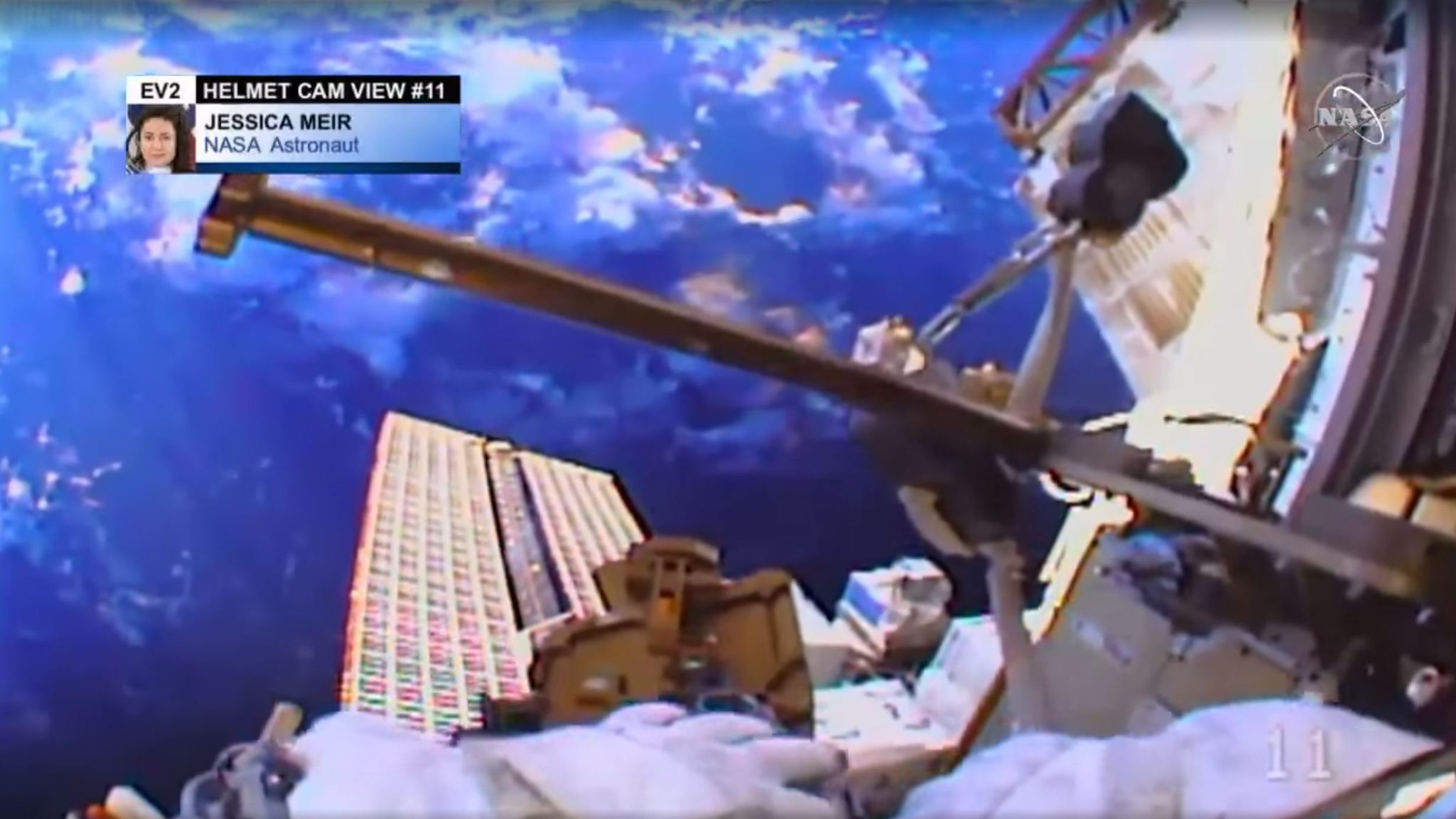The image captures a grainy photograph from what appears to be a launch center, showcasing an upward perspective into a blue sky scattered with fluffy white clouds. The foreground is dominated by metal supports and a tall building that seemingly reaches towards the sky. In the top right corner, the iconic NASA logo—a circular emblem with "NASA" written in red and a swooping ring around it—catches the eye. The top left corner contains a rectangular box with "EV2" in black lettering on a white background. Adjacent to this, on a black background, the words "Helmet Cam View 11" are displayed in white lettering. Below "EV2" is a small photograph of a woman with brown hair, identified as Jessica Meir, a NASA astronaut. Her name appears in a white box with black lettering, and directly below this, "NASA astronaut" is written in blue. The scene is filled with additional white machinery visible on the right and bottom edges, suggestive of part of a rocket or satellite structure being worked on, potentially for construction or repair purposes. The bottom right of the image also features the number 11 in white, tying back to the helmet cam view indication.